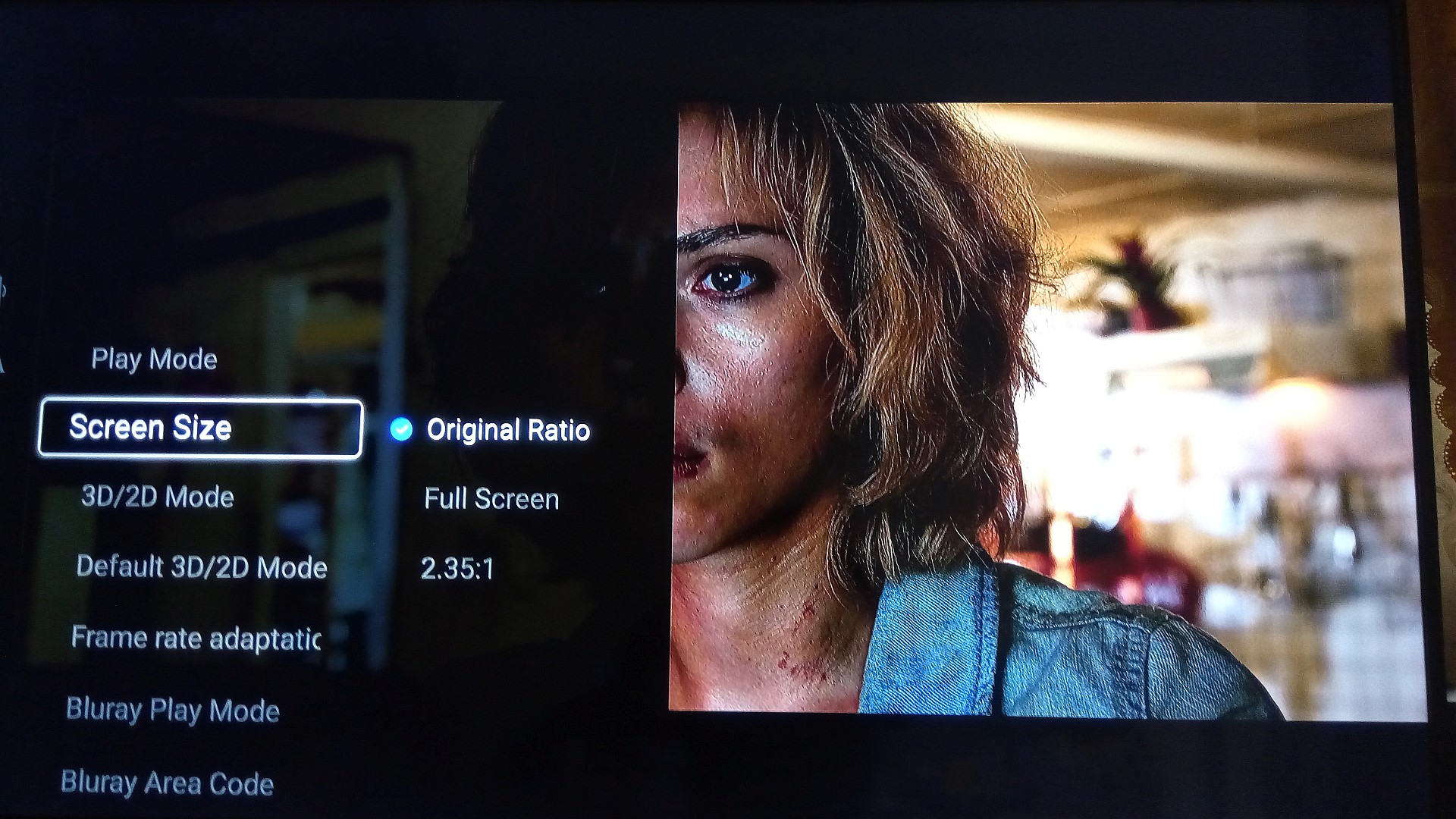The image shows a smart TV screen split into two sections. On the right side of the screen, partially obscured, is an image of a woman, possibly Scarlett Johansson, in a video or movie scene. Only the left half of her face and one shoulder are visible. She has long brown hair, appears to be looking forward, and is wearing a denim blue top. The background behind her is blurry, hinting that she might be standing on a street with some shops and a red car faintly visible. 

On the left side of the screen is the TV's settings menu against a black background with a slight reflection. The settings listed in white text include "Play Mode," "Screen Size," "3D/2D Mode," "Default 3D/2D Mode," "Frame Rate," "Blu-ray Play Mode," and "Blu-ray Area Code." The "Screen Size" setting is highlighted, and a sub-menu next to it offers options like "Original Ratio," "Full Screen," and "2.35:1," suggesting the user is currently adjusting these settings. 

Overall, the detailed scene juxtaposes the technical menu of the TV settings with the cinematic image of the woman, possibly from a movie, creating a contrast between technology and entertainment.